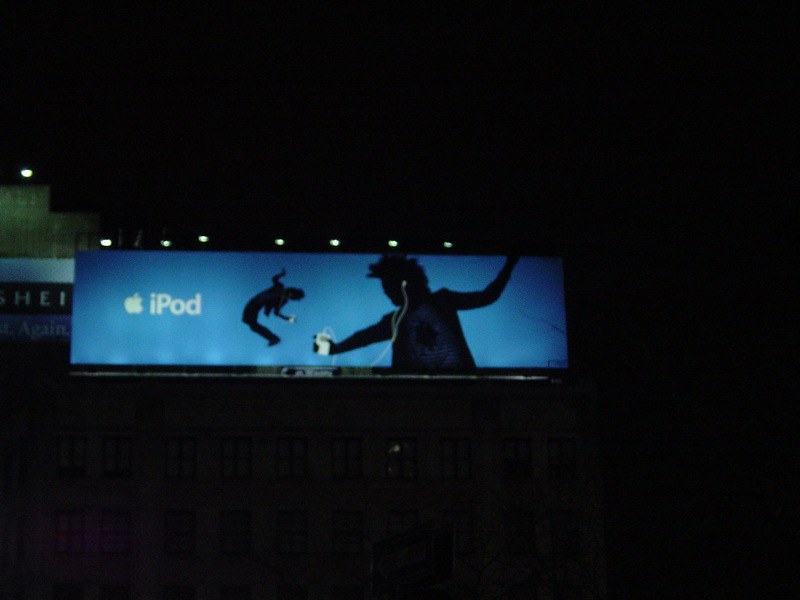The photograph depicts a large, brightly lit billboard against a pitch-black night sky. Positioned prominently in the middle, the billboard features an advertisement for an iPod with a striking blue background. To the left side of the sign, there is a white Apple logo followed by the word "iPod" in white letters. The image showcases two black silhouetted figures that appear to be dancing joyously. The first figure, positioned closer to the center, is in a dynamic pose with their head tilted back, one arm raised, and the other stretched downwards, holding a white iPod. White earbuds are visible, connecting the device to the figure's ears. To the right, another figure is depicted from the waist up, with their left arm outstretched, holding a white iPod. The cords from the earbuds run across the upper chest and into the figure's ears, complementing their lively posture with an arm raised in celebration. Above this billboard, seven evenly spaced lights illuminate the scene, emphasizing the vibrant advertisement. To the side, dark outlines of additional buildings or signs with partial letters "HEI" and "AGAIN" in white text can be seen, though mostly obscured by the darkness. The overall composition highlights the central Apple iPod advertisement against the contrasting blackness of the night.